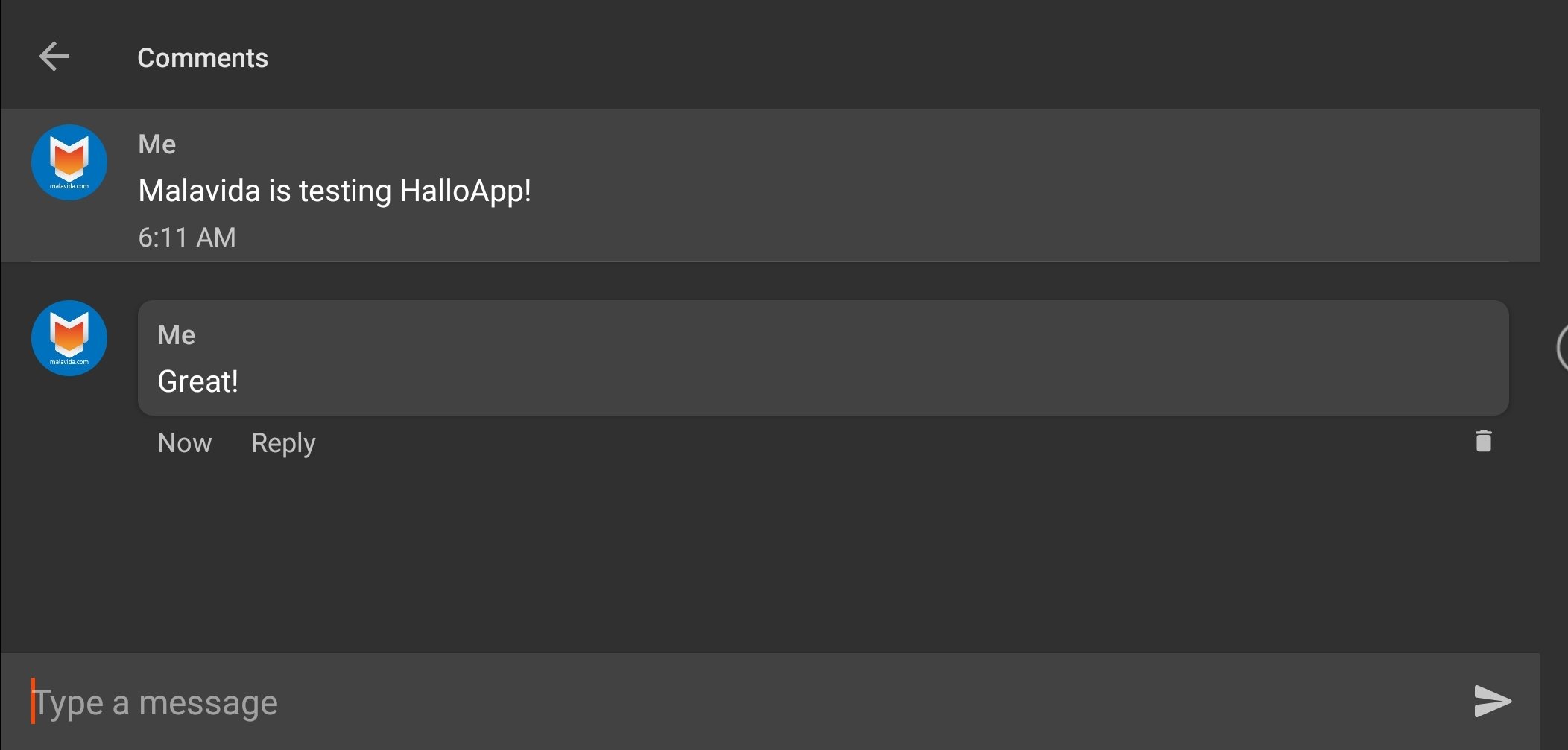In this image, the background is a solid black or dark grey color, creating a stark contrast for the white text. The texts represent a conversation or comments likely made on a social media platform or messaging app called HelloApp. The conversation starts with an initial comment from the user at 6:11 a.m. that reads, "Malavida is testing HelloApp." This is followed by a response from the user saying, "Great," which is marked as posted just now.

Towards the right side of the image, adjacent to the comments, there is a visible "delete" button, indicating the option to remove the message if needed. At the bottom of the image, there's a text field prompting the user with "Type a message," alongside a "send" button, where subsequent comments can be composed and sent. 

Overall, the image effectively captures a portion of a chat interface, showcasing the time-stamped, threaded nature of a conversation in HelloApp, supplemented with user options for message management and further interaction.